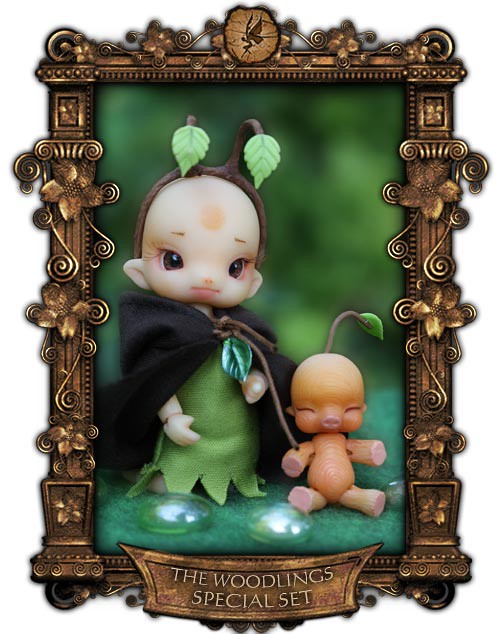The image is a detailed and enchanting digital drawing titled "The Woodlings Special Set," encased in an ornate, gold-bronze frame adorned with delicate floral and leafy motifs. At the bottom of the frame, the title is elegantly inscribed in white font. The backdrop of the illustration features a lush, green, leaf-like pattern, enhancing the whimsical forest theme.

Within this captivating scene, two whimsical dolls are prominently displayed. The doll on the left exudes an otherworldly charm with pointed ears and large, expressive brown eyes. She sports a crown-like arrangement of two green leaves stemming from her head, complemented by pink lips. Her attire consists of a flowing green dress beneath a mysterious black cloak, contributing to her ethereal appearance.

Beside her, on the right, stands a small baby doll of the same mystical species. This adorable figure has a single delicate stem sprouting from its head, ending with a tiny green leaf. Its peach-colored, wooden-textured body and pig-like nose lend it a unique and endearing look. Both dolls are positioned on a green, grass-like area adorned with small green marbles, enhancing the naturalistic, fairy tale ambiance of the piece.